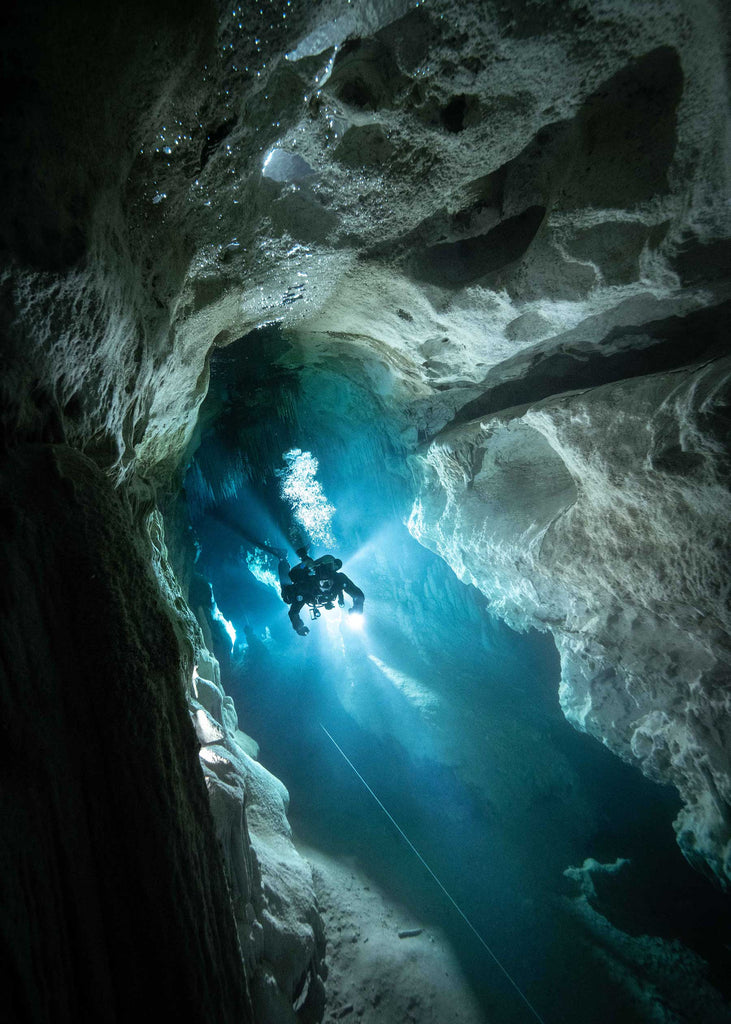This captivating photograph captures the thrilling, yet eerie experience of cave diving. A diver, clad in a thick black wetsuit and black fins, is seen exploring a dark blue, somewhat murky underwater tunnel. The diver, equipped with a large yellow oxygen tank and a breathing apparatus, holds a bright white light in their left hand, illuminating the shadowy surroundings dominated by white and gray rocks. Bubbles float above the diver's head, and a guide rope is visible at the bottom of the frame, extending into the ominous depths of the cave. The scene is framed by a narrow, tall crevice that curves from the mid-center to the bottom right, highlighting the tight and daunting nature of the underwater passage. The diver's isolation in this constricted, dimly lit space adds an element of spookiness to the image, enhanced by the subtle contrast between the light from the diver's lamp and the surrounding darkness.